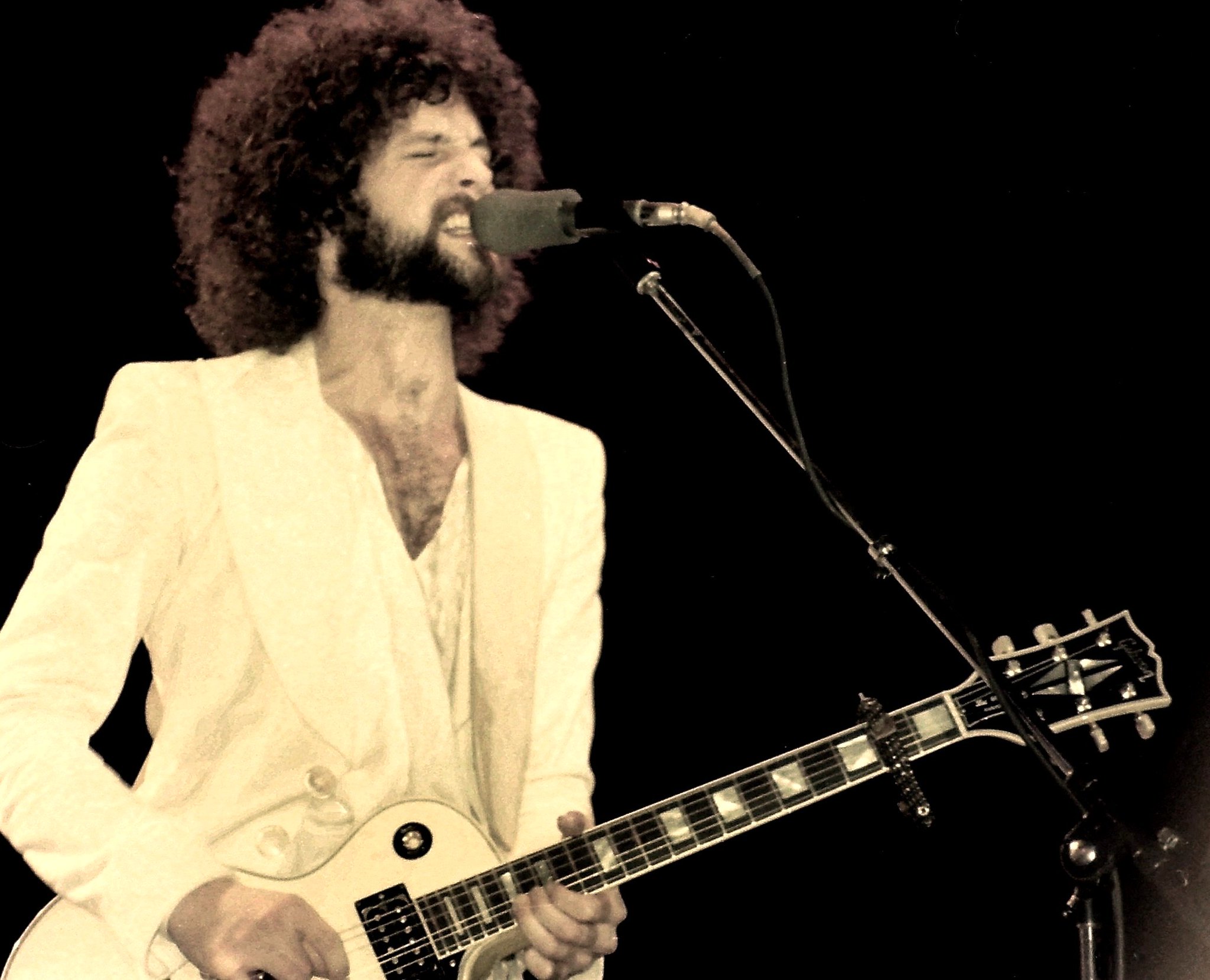In the image, a Caucasian man with a curly dark afro and brown mustache is passionately singing and playing a black and white electric guitar, which has more black on the neck and more white at the base. He stands in front of a metal, black microphone stand, leaning into the microphone which is covered with a sponge cover. His eyes are closed and his mouth is open, revealing his teeth as he focuses intently on his performance. The man is dressed in a white jacket over a v-neck t-shirt, exposing his chest hair, and he appears to have a dark vest underneath. He has a ring on his right hand, and there is a bar across the front of the guitar. The background is pitch-black, emphasizing the intensity and concentration of his musical moment.